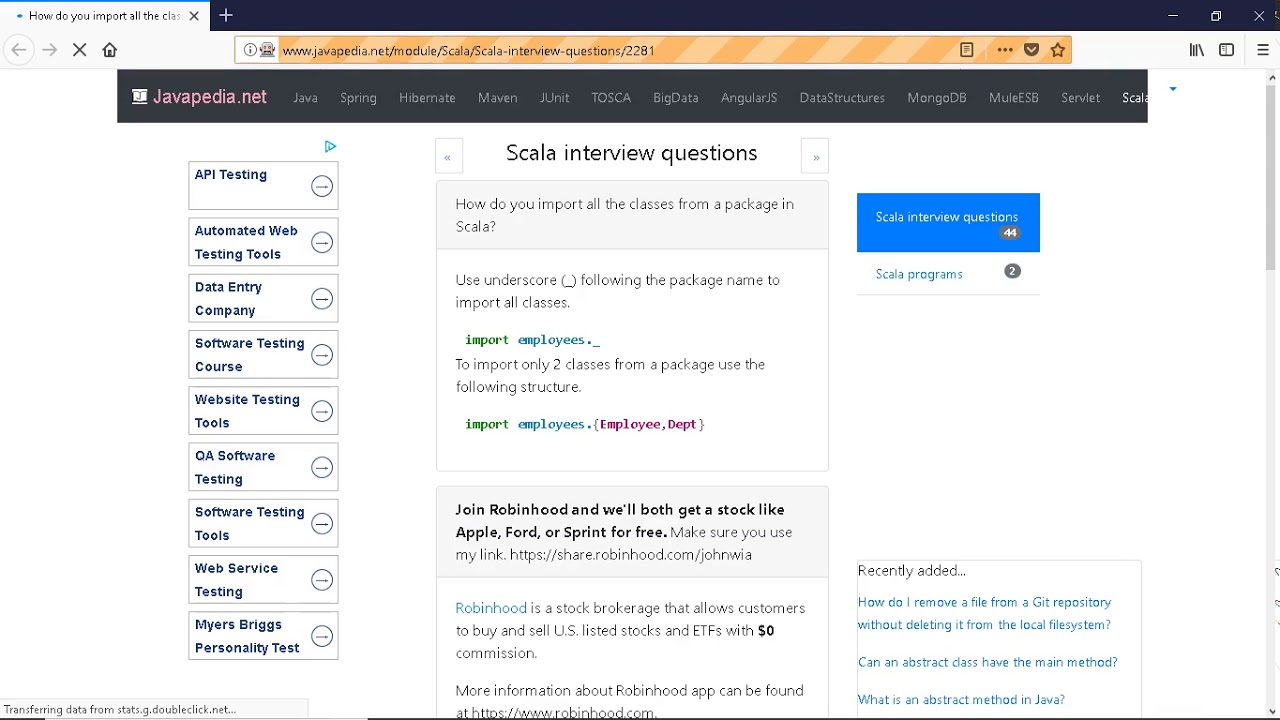Screenshot from the javapedia.net website. The site name, highlighted in pink, is prominently displayed at the top left corner. On the left sidebar, a navigable menu lists various pages, including "API Testing," "Automated Web Testing Tools," "Data Entry Company," "Software Testing Course," "Website Training Tools," "QA Software Testing," "Software Testing Tools," "Web Service Testing," and "Myers-Briggs Personality Test." Central to the image is a display featuring "Scala Interview Questions," with the first question asking, "How do you import all the classes from the package in Scala?"